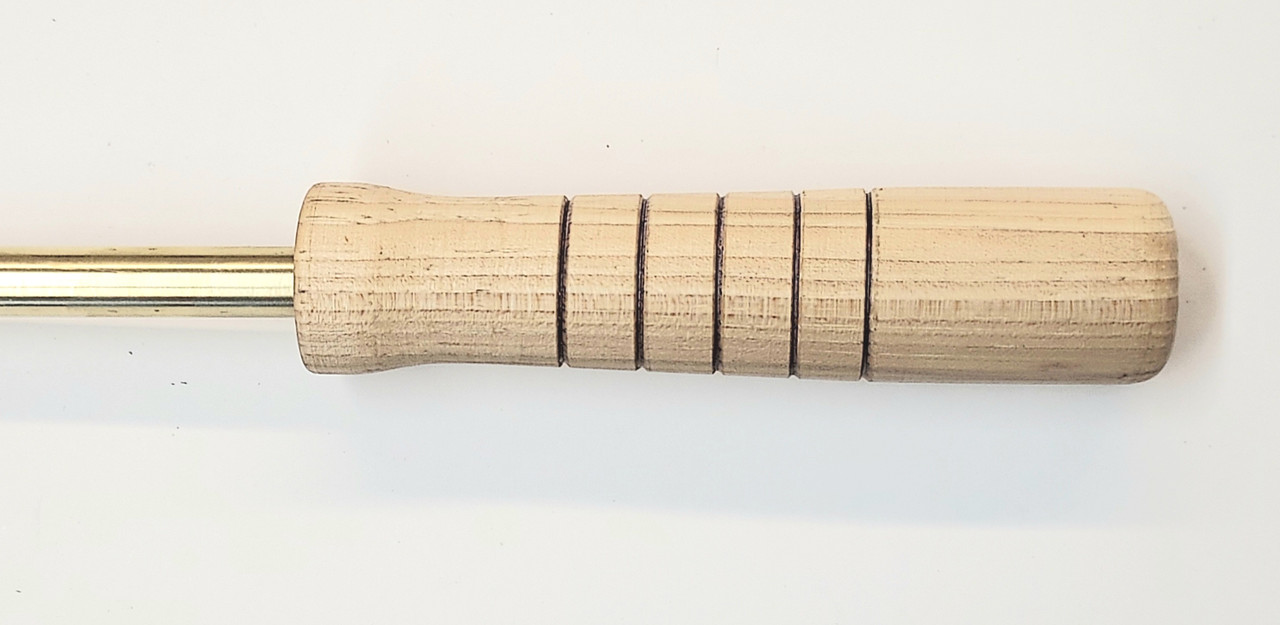This image features a light-colored wooden handle displaying prominent wood grain that runs horizontally. The handle is etched with five evenly spaced grooves, likely intended to enhance grip. Emerging from the left side of the handle, two narrow, golden metal rods extend out of the frame without revealing their endpoints. The photograph, likely taken indoors, presents the object on a white surface that bears small black speckles. The white background creates a slight shadow of the handle, adding depth to the scene. The object's exact purpose is unclear, but it could be part of a kitchen tool or another implement where a secure grip is essential.